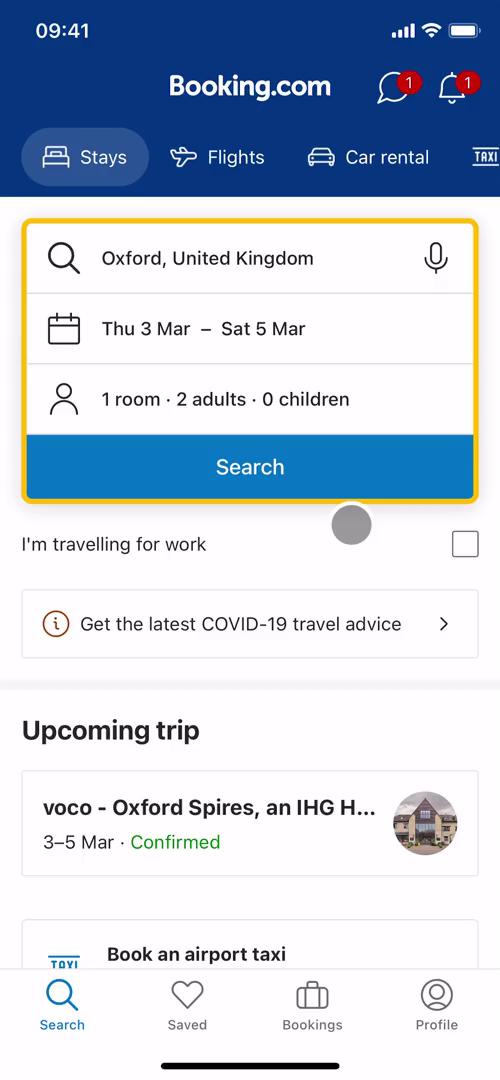In this image, we see a mobile app interface of a Booking.com webpage displayed on a smartphone. This is evident from the visible status bar at the top. The app's header is blue and prominently features the Booking.com logo. 

Beneath the header, there are navigation buttons for 'Stays' (likely for hotel reservations), 'Flights', and 'Car Rentals'. Below this navigation bar, there is a search bar filled in with "Oxford, United Kingdom." Directly under the search bar is a date range displayed as "Thursday, 3rd March to Saturday, 5th March," followed by an icon of a person indicating "1 room," "2 adults," and "0 children." There is also a search button that prompts, "I'm traveling for work."

Further down, there's an option linked to "Get the latest COVID-19 travel advice," followed by details of an upcoming trip. This section shows a small image of what is presumably a hotel named "VOCO Oxford Spires," noted to be part of the IHG chain, with a booking confirmed for the 3rd to 5th of March. 

At the bottom of the screen, there is a button for "Book an airport taxi," and a row of icons for 'Search,' 'Saved,' 'Bookings,' and 'Profile.'